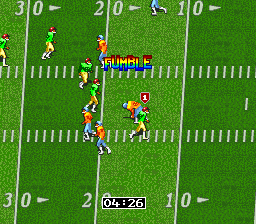A vibrant screenshot from a vintage American football video game, likely from the Sega Genesis or Super Nintendo era, showcases a moment of interrupted gameplay. The field features clearly marked white lines at 30-yard, 20-yard, and 10-yard intervals along with smaller ticks in between. Two teams are on the field: one donning green jerseys, yellow pants, and red helmets, while the opposing team sports orange jerseys, blue pants, and blue helmets. The word "FUMBLE" in eye-catching rainbow-colored text is emblazoned across the top of the screen, indicating a dropped ball. At the bottom, a timer reads 4 minutes and 26 seconds remaining in the quarter. Ten players are visible, with five from each team dispersed across the field in anticipation of the next play.